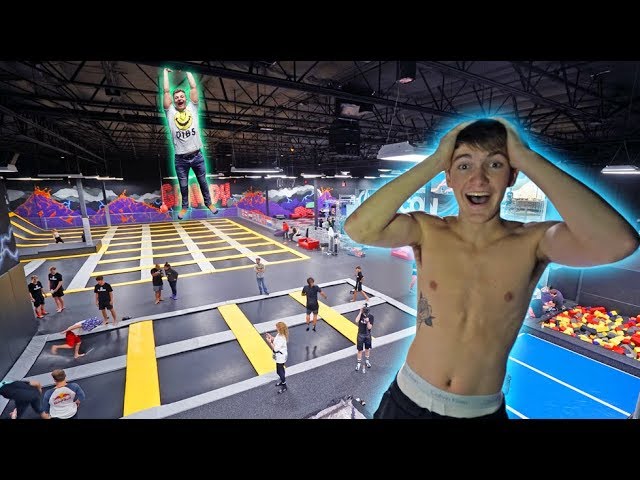In this vibrant and dynamic image, likely intended as a YouTube thumbnail or online video preview, we see the lively interior of an indoor trampoline park. The bottom right corner features a shirtless boy glowing in blue, wearing white underwear and black shorts, with his hands on his head, eyes wide, and mouth open in a mix of surprise and excitement. Above him to the left, another man, glowing in green and wearing a white tank top and dark pants, hangs photoshopped from the rafters, arms raised. The trampoline park itself has sectioned areas of dark, shiny black floors marked with yellow strips, foam pits, and trampolines. A wall painted with volcanoes and a foam pit occupy the lower right section, while various people enjoy the park throughout. The upper part of the image includes part of the park's ceiling. The man hanging from the rafters sports a shirt with the text "dibs," drawing attention to his playful and exaggerated pose. The overall palette of the image includes hues of blue, peach, white, black, yellow, purple, and orange, adding to its colorful and engaging composition.